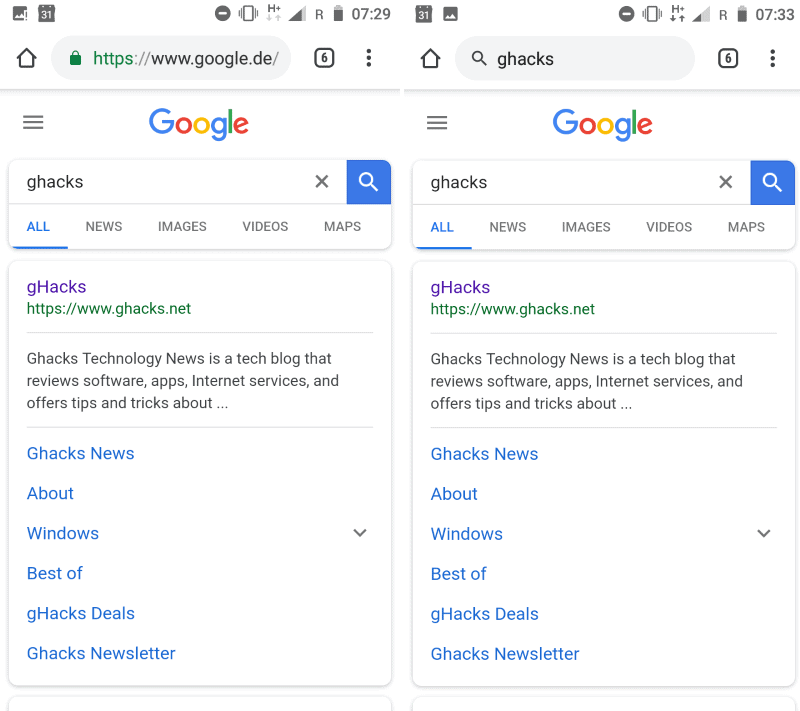This image, captured from a cell phone, displays two Google search results side by side, seamlessly combined into a single picture. The uniform white background spans across both halves, giving the impression of a cohesive interface despite the two distinct searches. 

On the left side, the browser's URL bar shows "https://www.google.de/", hinting at a search conducted on the German version of Google. Notably, a lock icon, indicating a secure connection, is present beside the URL. Below the URL bar, the Google search area is clearly visible with the multicolored Google logo and the search term "GHACKS." 

On the right side, the URL bar interestingly displays "GHACKS," written as a single word, but lacks a typical URL format, suggesting it may be a custom label or identifier rather than a standard web address. The search interface mirrors the left side with the familiar Google layout, including the same multicolored logo and search term.

Under both search bars, a menu allows for further navigation with options like "All," "Images," "Videos," and "Maps." In the search results area, a highlighted green clickable link reads "HTTPS," indicating a secure webpage. Below this, a snippet describes "GHACKS technology news as a tech blog that reviews software apps, internet sources, and other tips and tricks about..." with text trailing off into an ellipsis, suggesting more content continues below.

The bottom segment of the phone displays additional search results and information, maintaining consistency with the rest of the image.